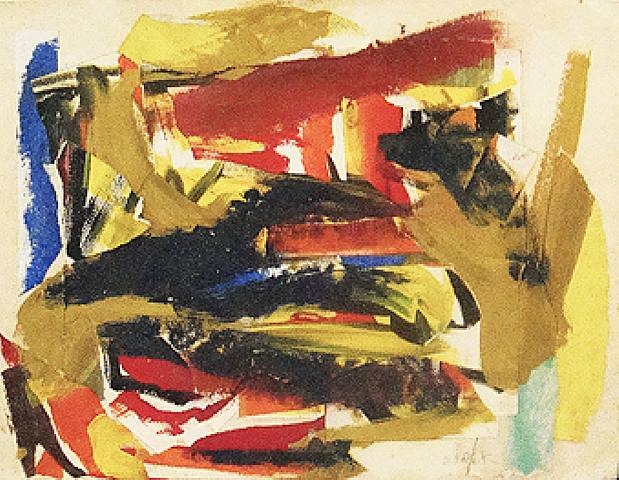This is an abstract or modern art painting on a white, almost off-white canvas background, characterized by large, thick, and haphazard brushstrokes. The painting prominently features various shades of gold and yellow, accented by lighter golds and yellows that create a dynamic, curving motion across the canvas. Bold black brushstrokes are strategically placed, primarily in the middle and along the edges, adding depth and contrast. Dominating the center are wide, striking swathes of dark blood red, which transition to a more orange-red hue towards the bottom. Interspersed among these colors are two bright blue spots; one is located in the middle of the design, while another bright blue slash runs horizontally on the upper left side, extending towards the middle. Additionally, there are scattered patches of blue within the central area. The composition also includes vertical strokes of orange and an irregular black shape in the center, reminiscent of a lobster, surrounded by the dominant red, gold, and yellow hues. The intricate interplay of these bold colors and strokes creates a vibrant, chaotic yet harmonious visual experience.